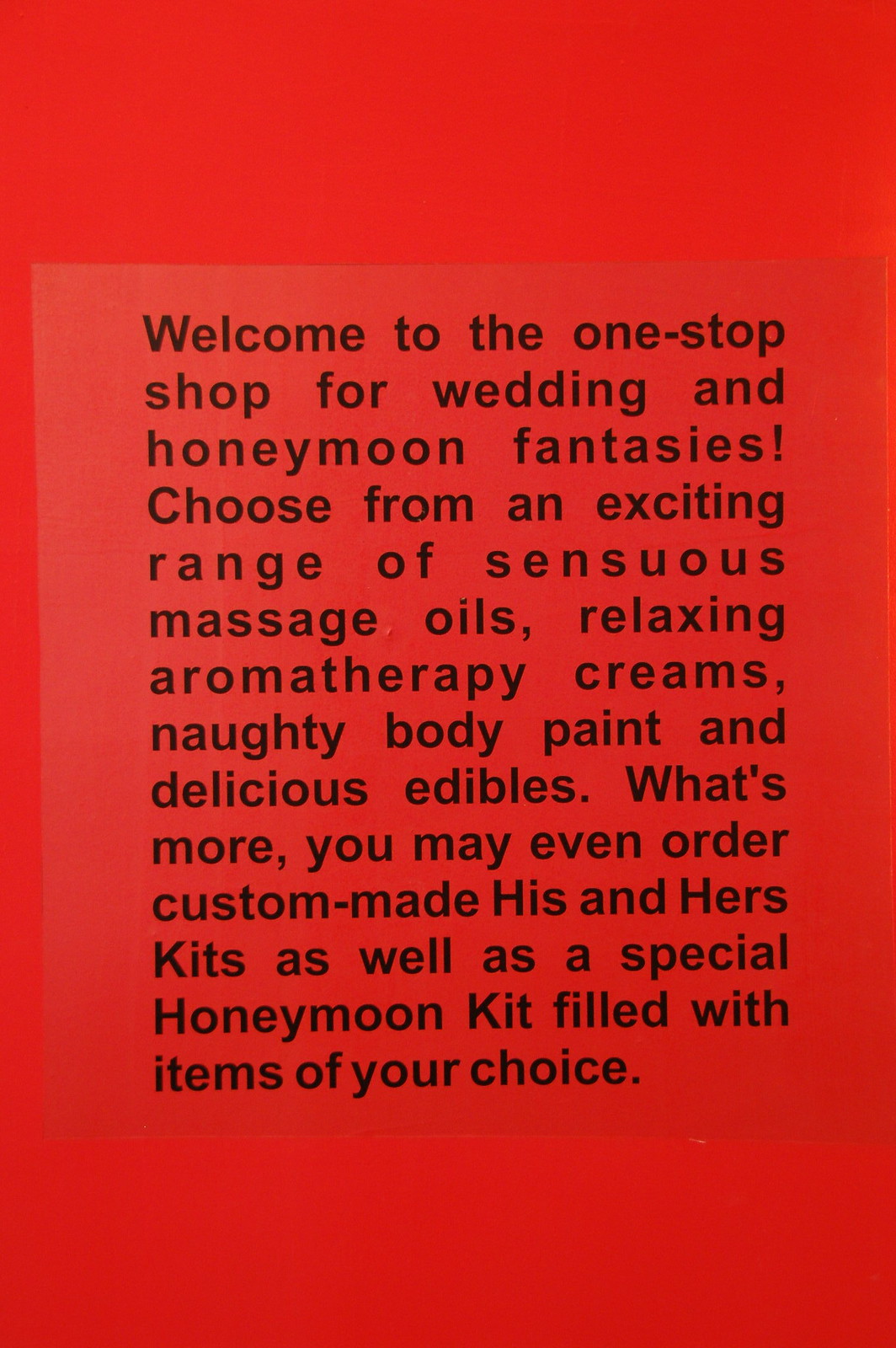The image is a photograph of a vertical rectangle sign featuring black text on a solid red background. The text is centrally aligned and appears slightly tilted to the left. It reads: "Welcome to the one-stop shop for weddings, wedding and honeymoon fantasies. Choose from an exciting range of sensuous massage oils, relaxing aromatherapy creams, naughty body paint, and delicious edibles. What's more, you may even order custom-made his-and-hers kits as well as a special honeymoon kit filled with items of your choice." The text seems to be printed on a clear piece of plastic, allowing the vibrant red background to be visible through it. There is additional red blank space both above and below the text, emphasizing the message in the center.